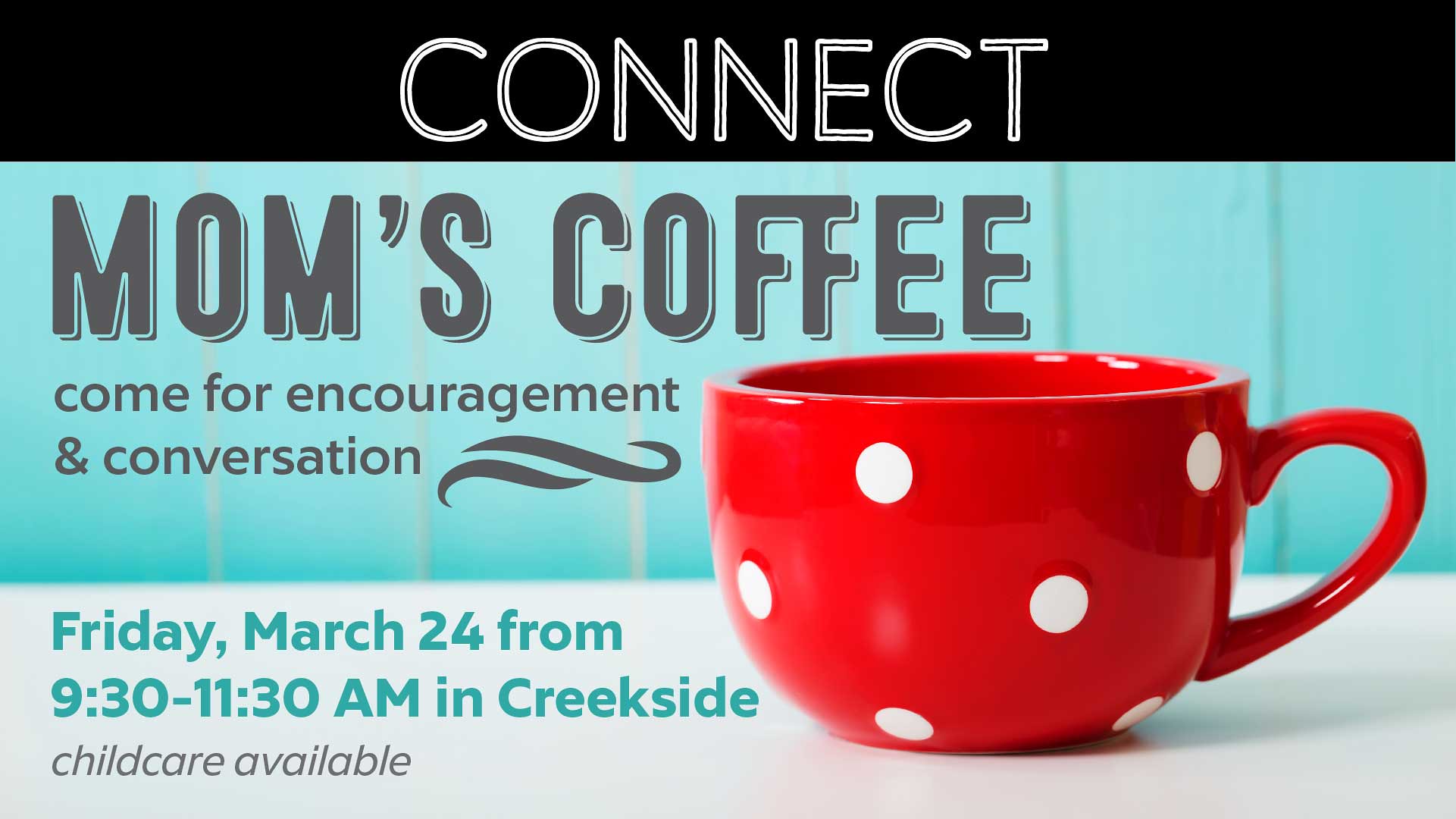This flyer, targeted towards moms, features a prominent black border at the top with white text that reads "Connect." Beneath this, a turquoise blue section contains gray text stating "Mom's Coffee: Come for Encouragement and Conversation," accompanied by a distinctive swoosh design. To the right of the text is a red coffee cup with white polka dots. The bottom portion of the flyer has a gray band resembling a table, which provides event details in greenish-gray text: "Friday, March 24th from 9:30 to 11:30 a.m. in Creekside." Beneath this, it indicates "Child Care Available." The background of the image is a light blue seafoam green, giving the flyer a cohesive and inviting aesthetic.